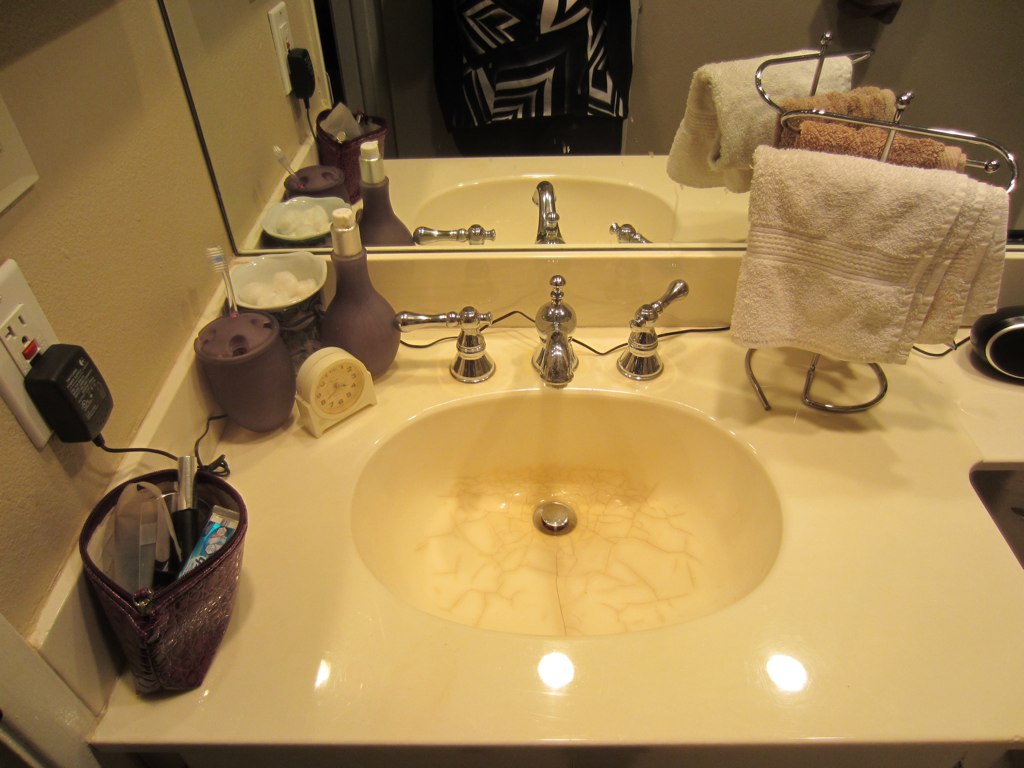In this photograph, we observe a moderately worn and cracked bathroom sink, accompanied by a silver faucet and handles. The sink rests on an ivory-colored countertop, which continues into a vanity. At the top of the image, a mirror spans the width of the sink, reflecting the entire scene as well as the image of a person wearing a shirt with a geometric design. 

To the left side of the sink, three brown containers of varying shapes are positioned. One container resembles a light bulb, another is round and holds cotton balls, and the third is also round but has a clear toothbrush standing upright in it. In front of these containers sits a white timer. 

Further left, near the front of the counter, there is a makeup bag brimming with various cosmetics and toothpaste. Above this section of the sink, a metal towel rack is affixed to the wall, from which hang two towels: a tan towel in front and a light brown one behind it.

Overall, the picture captures a detailed snapshot of a lived-in bathroom sink area, complete with personal hygiene and grooming items.